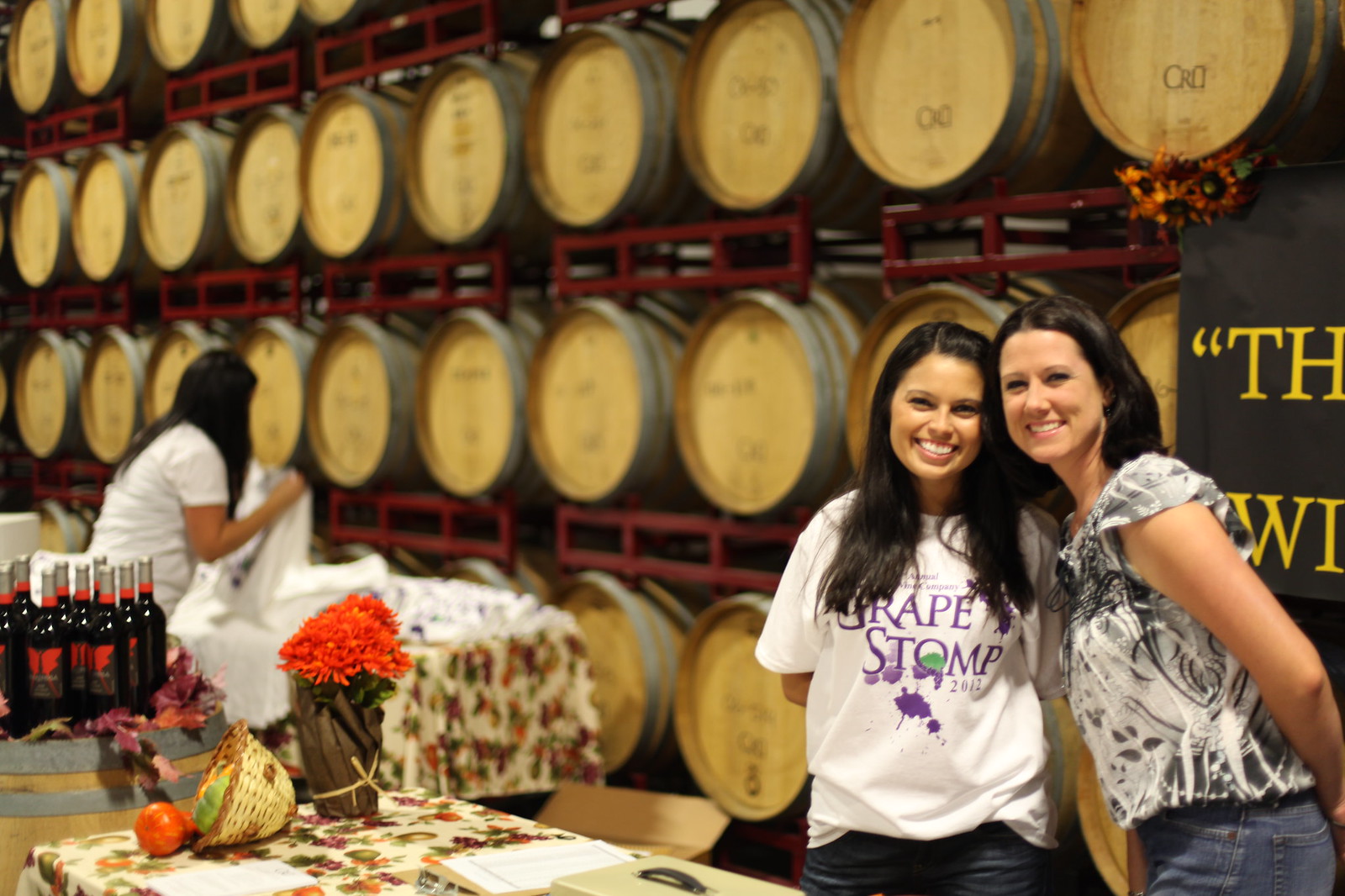This detailed photo captures a lively scene at a winery, specifically during the GrapeStomp 2012 event, as indicated by the purple text on the white t-shirt of one of the women. The image features three women amidst a backdrop of wine barrels and vibrant colors including purples, beige, tan, whites, blues, light brown, orange, and black.

Prominently positioned in the bottom right corner are two women. The woman on the left, possibly of Indian or Latina descent, has long dark hair and wears a white t-shirt with "Grape Stomp 2012" in purple letters, paired with jeans. Beside her is a white female with dark, shoulder-length hair, donning a white and black blouse and jeans. They stand near a table covered with a floral pattern cloth, adorned with a vase of bright orange flowers, a tipped-over basket with a pomegranate or apple, a cash box, a clipboard with papers, and an assortment of books and flowers.

In the left middle background, a third woman, whose face is obscured, is engaged in folding linens. She has very dark hair and is also wearing a white t-shirt. The wine barrels in the background, organized in racks, transition from being blurry on the left to more clear on the right, each topped with light wood and silver rims. A wine barrel adjacent to the table is stationed with about a dozen wine bottles, identifiable by their black bodies with red and gray labels.

This dynamic image captures the essence of a bustling winery event, with an array of detailed elements and a harmonious blend of colors and activities.